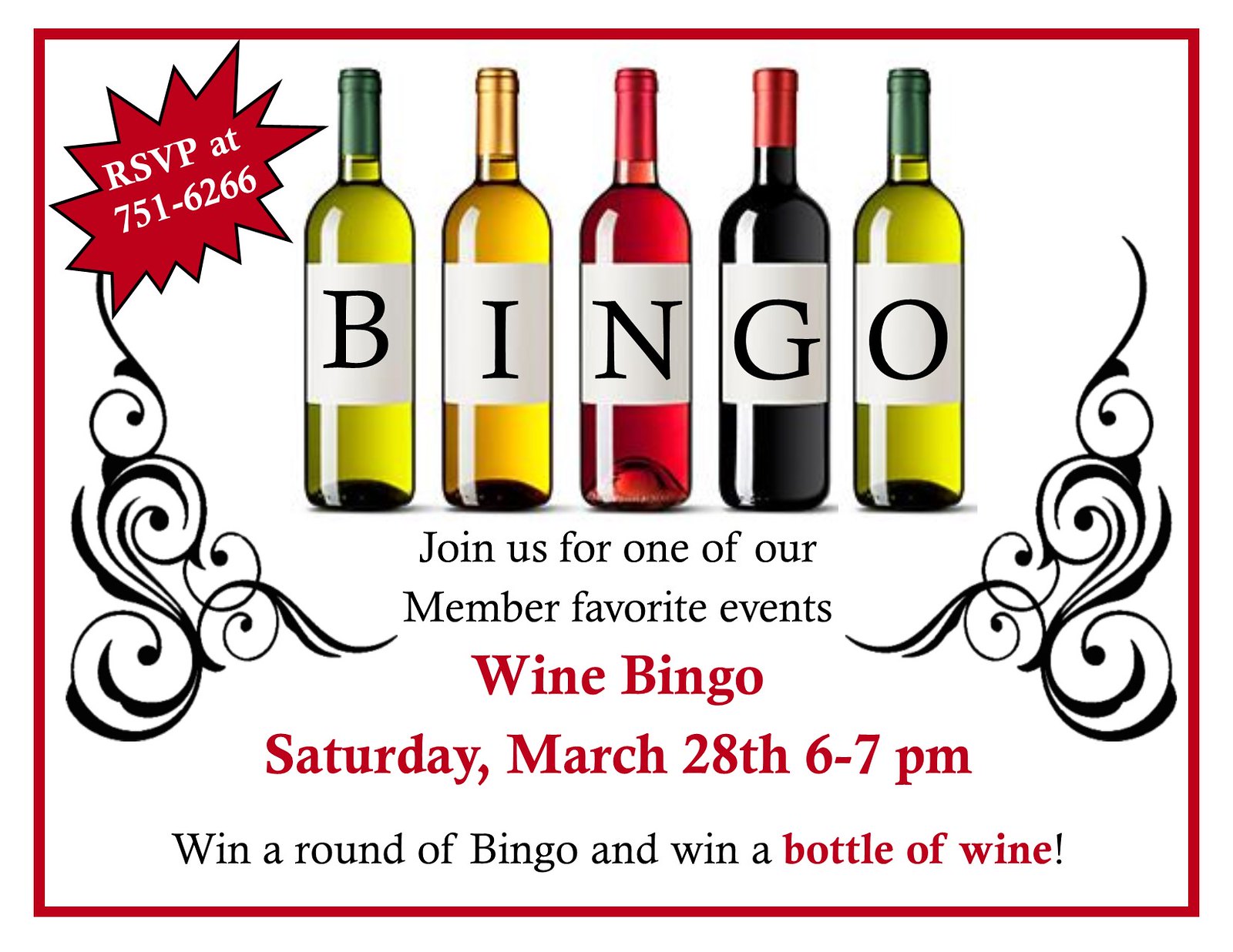The image is a computer-generated ad or invitation with a white background and a prominent red rectangular border. In the top left corner, there is a red, burst-shaped icon featuring white lettering that reads "RSVP 751-6266." Adjacent to this RSVP icon are five illustrated wine bottles in various colors: green, gold, red, black, and another green. Each bottle's label displays a letter, collectively spelling out "BINGO."

Below the wine bottles, the text invites viewers to join a favorite member event: "Wine Bingo." The invitation details are clearly stated in different font colors: "Join us for one of our member favorite events, Wine Bingo, Saturday, March 28th, between 6 and 7 p.m." It further entices participants with the promise, "Win a round of bingo and win a bottle of wine," with "bottle of wine" highlighted in red font. Black decorative swirls adorn either side of the image, adding a touch of elegance.